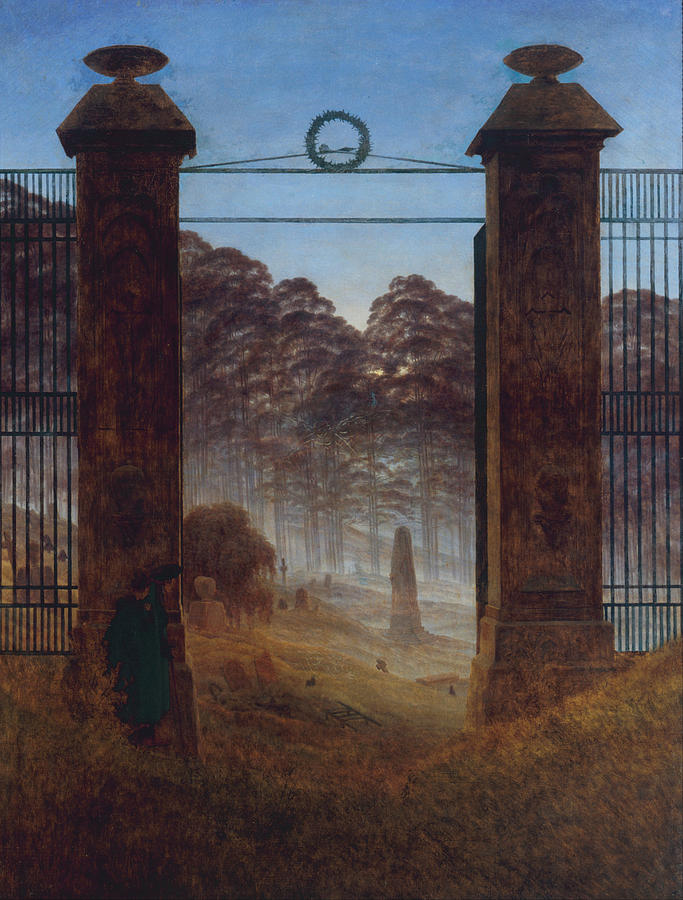The image is a detailed painting of an old, neglected cemetery viewed through an open gated entrance. The entrance is flanked by two tall, rectangular stone pillars about a story high, each supporting ornate metal gates. A wreath-shaped object adorns the top space between the pillars. In front of the entrance, the ground is a mix of green, black, pink, and yellow hues, suggesting grass and various foliage. 

Inside the gates, the landscape reveals a rolling hill that descends from left to right, adorned with decayed tombstones and crosses. Some gravestones are rounded, and there's a small stone monument amidst the overgrown grass and an uncared-for bush. In the foreground, two darkly-clad figures stand peering into the cemetery, adding to the eerie atmosphere. 

Behind the cemetery, a dense cluster of tall trees stretches across the scene, with a sky above that is a deep blue with subtle hints of clouds. The time appears to be around dusk, as the setting sun casts long shadows and a soft, diffused light over the entire scene, further highlighting the desolate and abandoned state of the cemetery.